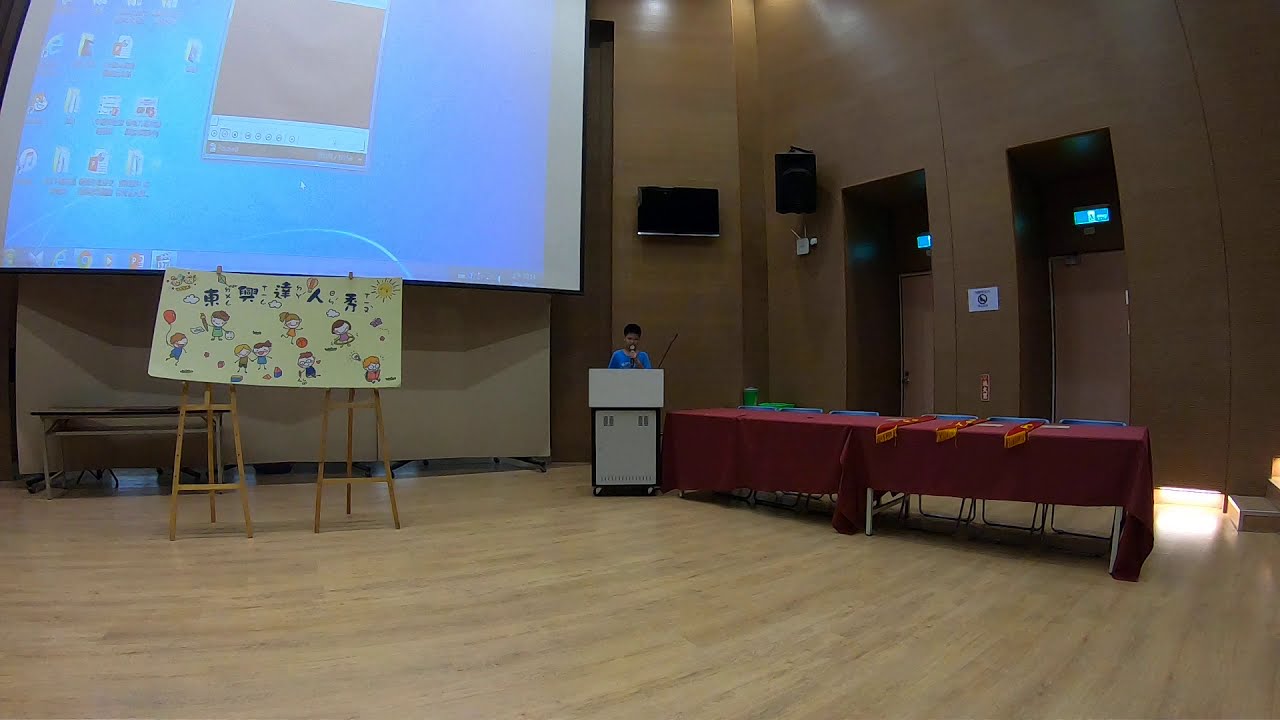The image depicts an indoor auditorium with a light brown wooden floor. The far wall is dark brown, featuring two light brown doors, each adorned with a green, backlit rectangular sign. In front of these doors, there's a setup of two tables, pushed together and draped in burgundy tablecloths, with six chairs featuring silver legs and blue seats arranged behind them. To the left of the tables stands a white podium with black trim, behind which a person in a light blue shirt is speaking into a black and gray microphone. 

To the left side of the image, a large screen projects the contents of a computer's home page, indicating a presentation in progress. Below the screen, a yellowish poster board with various childlike cartoons, including images of a kid holding a balloon and another kicking a ball, is propped up on wooden easels. The setting suggests the room could be used for school events or public gatherings, giving a warm and structured ambiance perfect for a formal presentation or meeting.